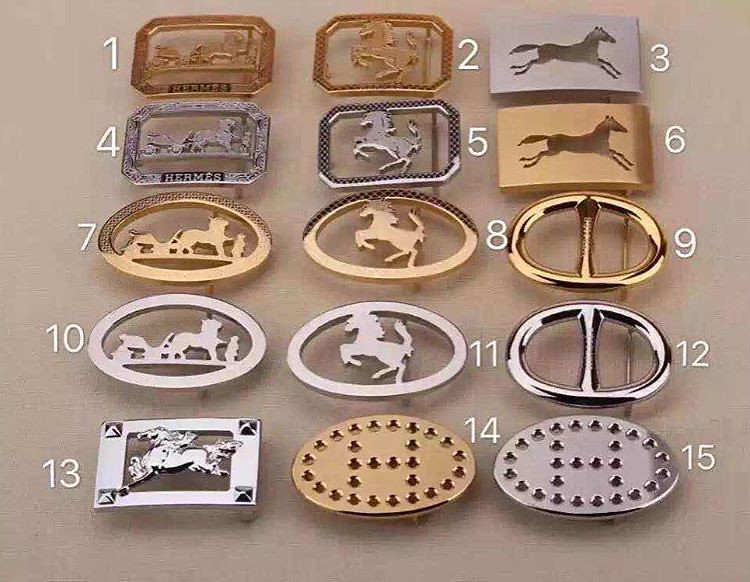This detailed, grainy studio photograph showcases a collection of 15 distinct belt buckles, meticulously arranged in a grid of three rows and five columns. Each buckle is labeled with a white number placed alongside it. The buckles are crafted in various metallic hues, predominantly gold, bronze, and silver, and display diverse shapes—some are round while others are square. A majority of the top twelve buckles bear intricate silhouettes of horses, either prancing, running, or drawing carts, with refined details highlighted subtly at the top of the image. The top six buckles, primarily square with trimmed corners, exhibit black horse silhouettes set against gold and silver backgrounds. The middle six are more elliptical and feature hollow designs with prancing horse motifs. In contrast, the bottom three buckles, including numbers 9 and 12, are simpler, adorned with solely a single vertical line or spikes, devoid of horse imagery. The assortment appears to be methodically photographed, likely intended for catalog display or ordering purposes.